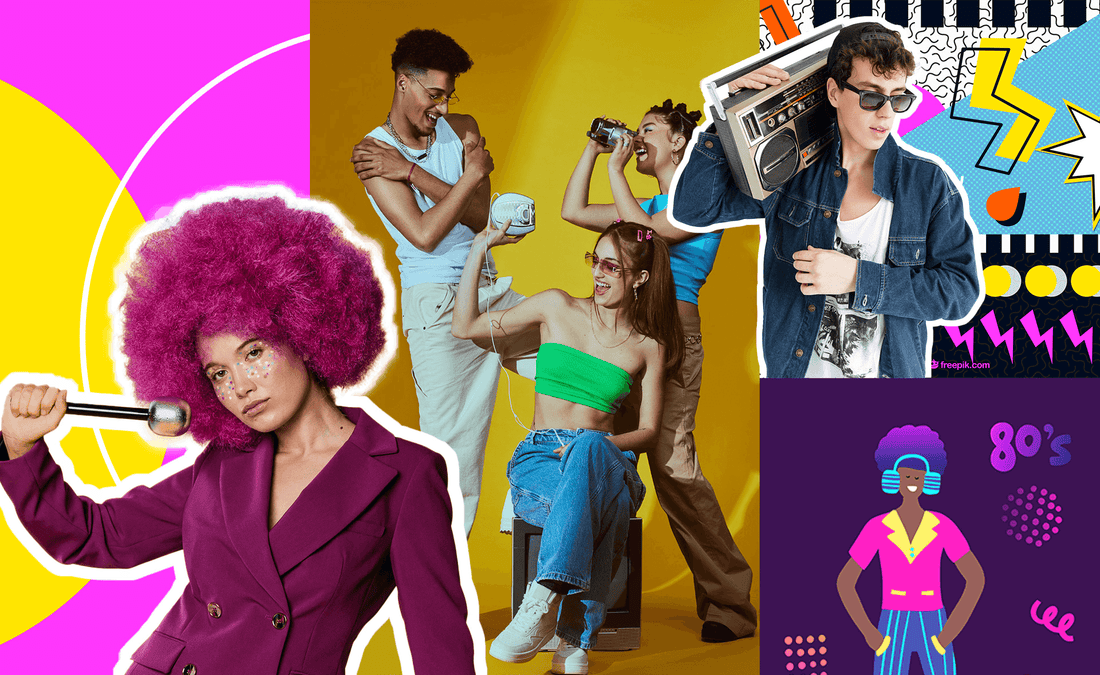This vibrant pop art collage exemplifies a fusion of 1980s and 1990s aesthetics across four distinct panels. On the left, a young woman with a striking, burgundy rose-colored Afro stands out, wearing a buttoned-up burgundy blazer and holding a black-handled microphone tipped with gold. Glitter and polka dot stickers decorate her nose and under her eyes as she stands against a neon backdrop of pink and yellow, outlined in white to enhance her prominence. 

The center panel showcases three individuals exuding a late 90s fashion vibe. Seated in the foreground is a smiling girl with long brown hair, adorned in rose-colored sunglasses, a bright green tube top, and wide-bottom blue jeans. Flanking her are a guy in a white tank top and jeans with his arms crossed, and another girl aiming a handheld camcorder. This girl wears a blue T-shirt and khakis, encapsulating the 90s youth culture beneath a vivid yellow background.

In the upper right, the scene shifts to an 80s motif featuring a young man with a denim jacket, white T-shirt, and Ray-Ban sunglasses. His backwards baseball cap and boombox perched on his shoulder epitomize the era, complemented by dynamic graphics including white stars, exclamation points, and splashes of turquoise, hot pink, and yellow.

The lower right portion diverges into a vector illustration of a black woman with a purple and pink Afro. She wears cyan headphones and a bright pink shirt with a neon yellow collar, her hands casually resting in her pockets. Behind her, the word "80s" forms a bold backdrop in purple, conclusively tying together the collage's nostalgic homage to these iconic decades.